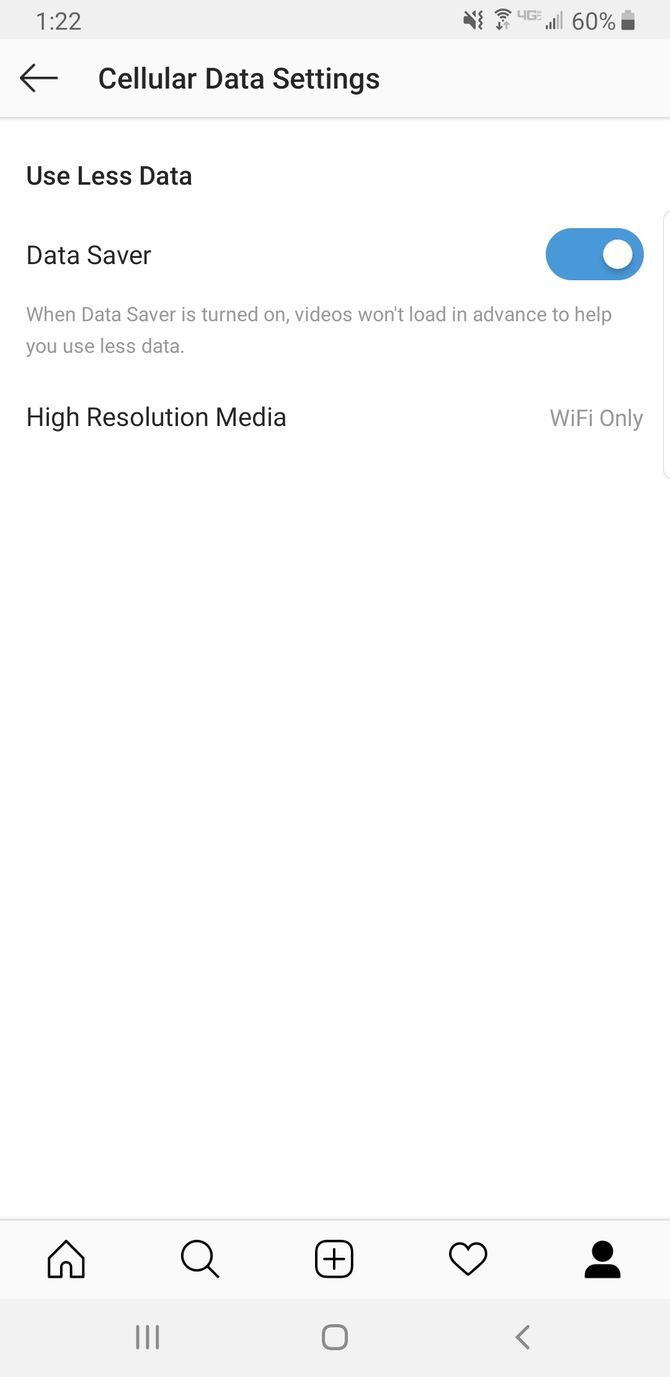In this image, a cell phone is displaying a settings page focused on data usage options. The status bar at the top clearly indicates it's a cell phone, featuring icons from left to right: the current time, volume control, Wi-Fi signal, network signal, and battery meter.

Directly below the status bar, there's a header labeled "Cellular Data Settings" accompanied by a back arrow, allowing easy navigation to the previous screen. 

The next section is titled "Use Less Data" which is followed by the "Data Saver" option, showing a toggle switch set to 'On'. An explanatory note underneath clarifies that with Data Saver activated, videos won't preload, conserving data usage. It also specifies that high-resolution media is restricted to Wi-Fi connections only.

The layout of the page is minimal and straightforward, clearly designed to inform users about their data-saving configurations and to provide easy access to adjustments.